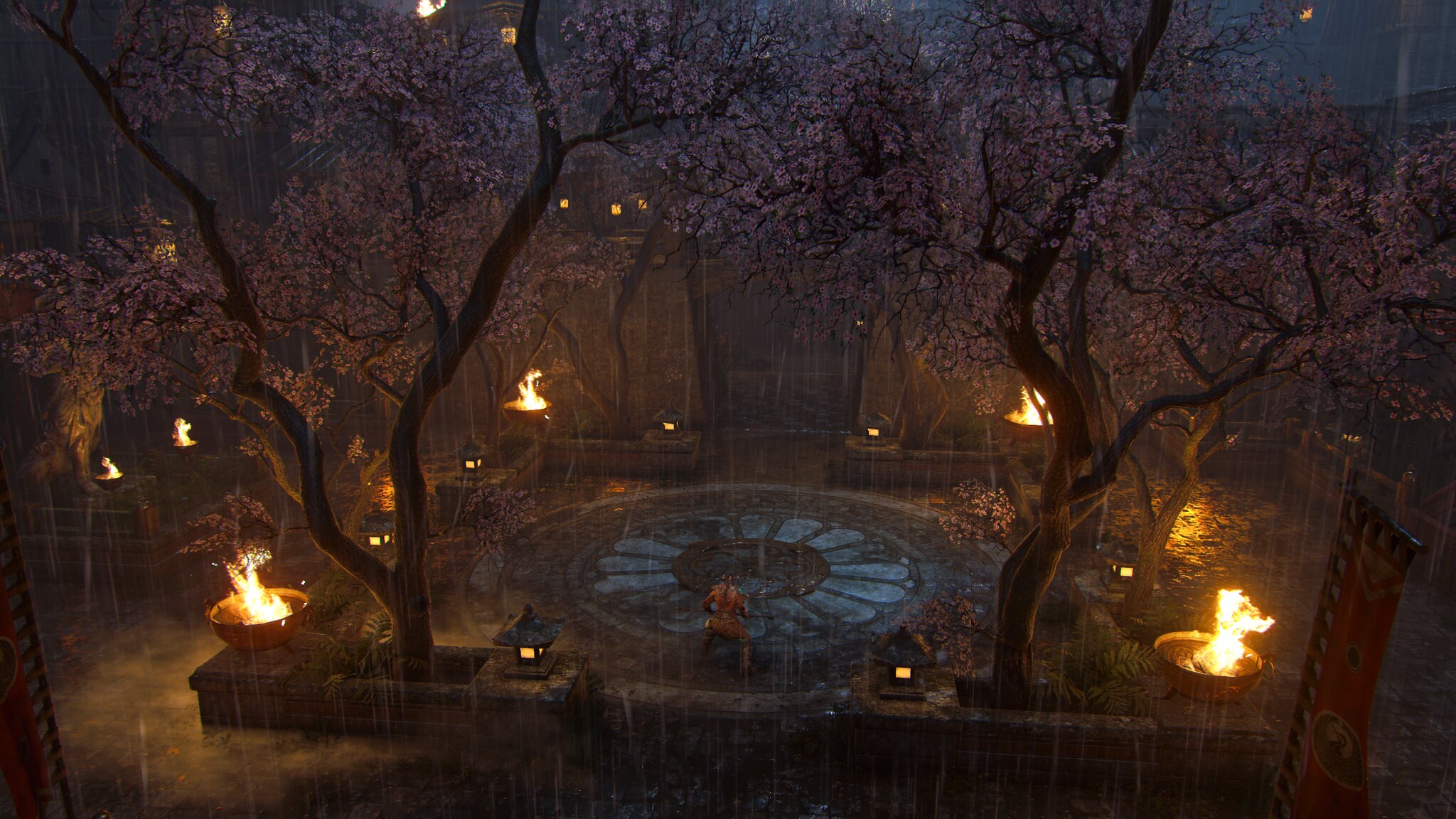The image portrays an aerial view of a serene, gated garden that exudes the tranquil aesthetics of a Japanese garden. Encased by a stone wall, the garden's layout features a meticulously designed platform in the shape of a raised square. At each of its four corners, there are fire pans, adding an intriguing element to the scene. The ground within the raised area showcases a unique pattern reminiscent of old-fashioned tombstones, arranged such that their pointed tops create a circular formation, with the bases converging at the center. This design element, coupled with the overall symmetry, evokes the image of a flower with a dark center. Surrounding the raised square, trees are in full blossom, contributing to the garden's serene atmosphere. There's a subtle reflection of light on water visible to the right, enhancing the peaceful setting. Amidst the captivating details, there appears to be a figure standing in the middle of the platform, further adding to the intriguing ambiance of this beautifully crafted garden scene.